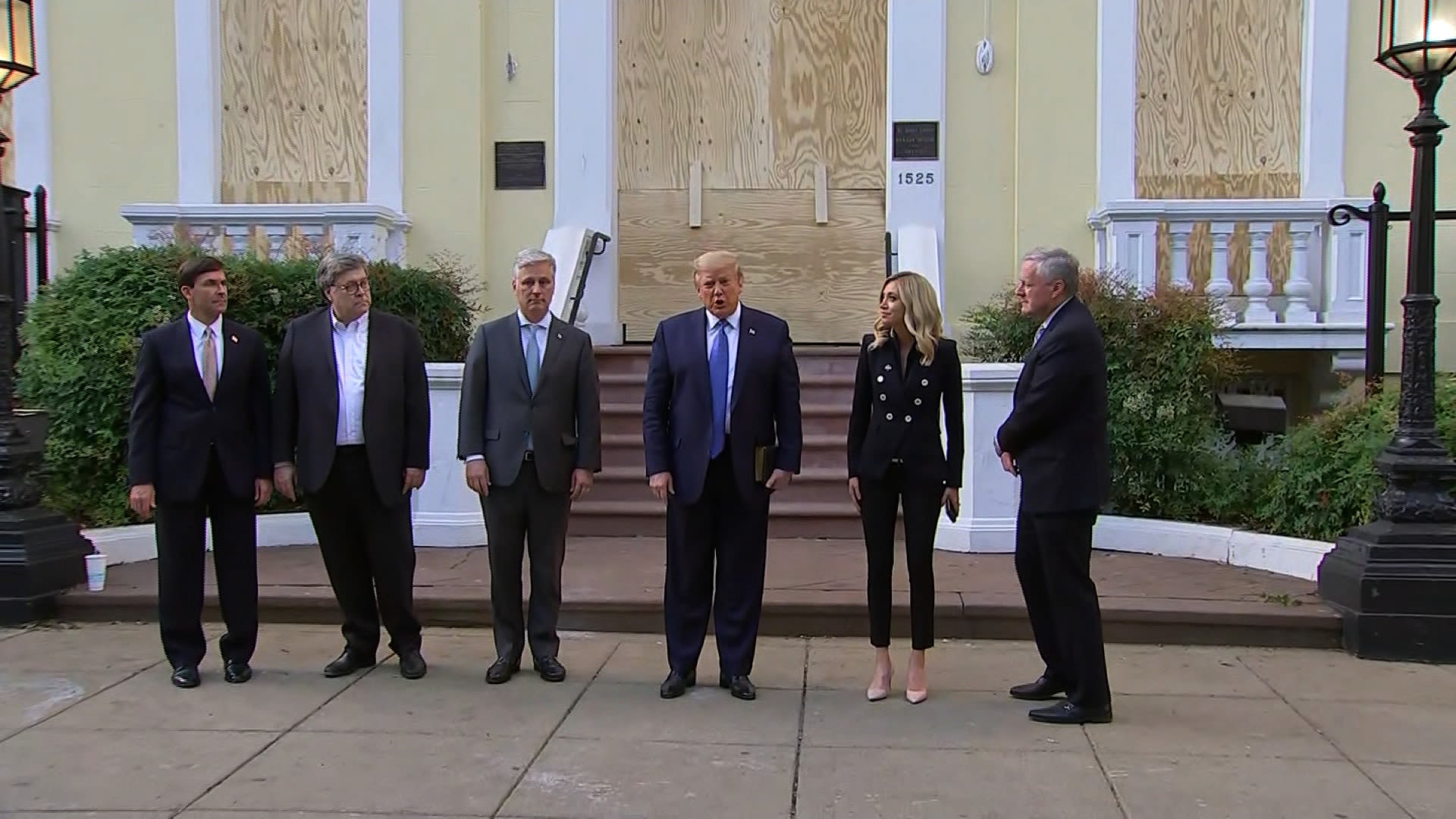This image features a group of six people, including Donald Trump, standing in front of a yellow building with white trim, which appears to be a church and is notable for having its windows and doors boarded up with plywood, possibly following the George Floyd riots. The ground beneath them consists of large square concrete slabs. The building is marked with the number 1528. Two lampposts are visible on either side of the group, with green shrubs and other vegetation adding some natural elements to the scene.

Donald Trump, positioned in the middle, is distinct with his blue suit and tie. He is holding a book. To his right stands the only woman in the image, recognizable by her blonde hair and black suit, which features golden buttons on her torso. She, too, is holding something in her hand. The other men in the group, including a possible identification of Steve Bannon and George Barr, are dressed in dark blue or black business suits with white button-up shirts and dress shoes. One man on the right side of the image is turned to the side, looking off to the left. The image is taken during the daytime.